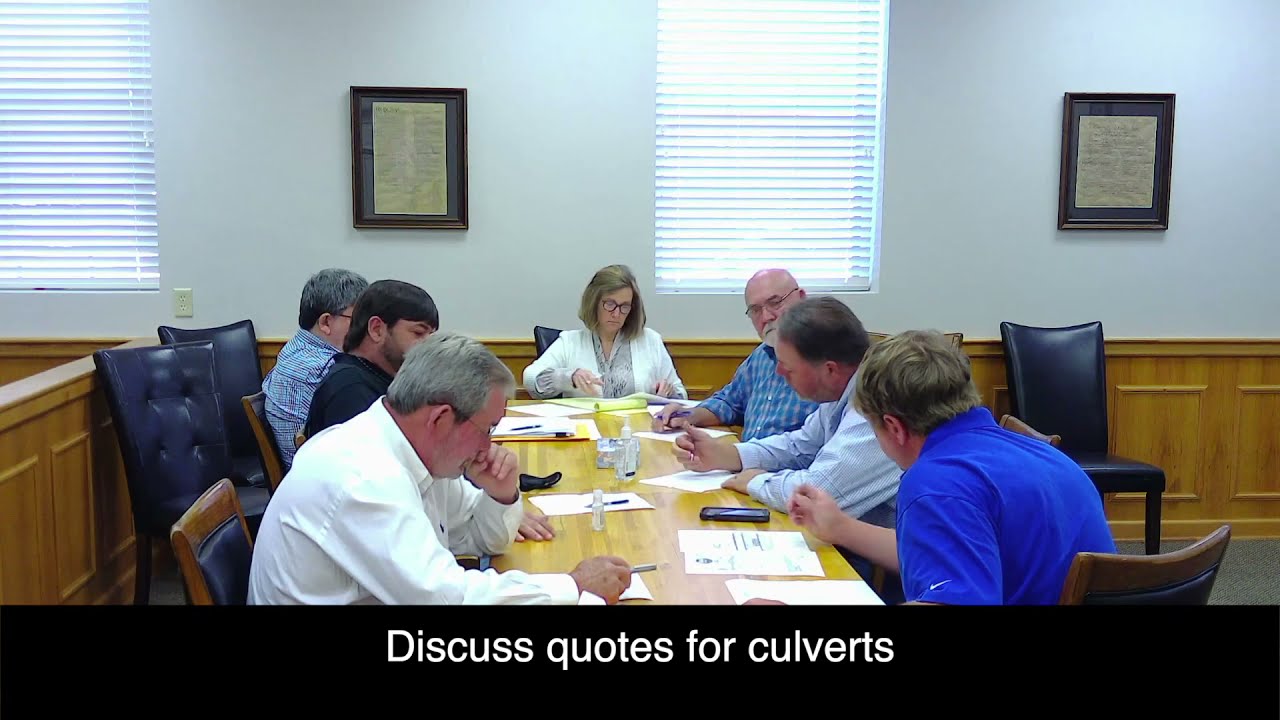In a plain boardroom, seven people are seated around a large, light wood tan rectangular table, deeply engrossed in discussing quotes for culverts. The man at the bottom right is wearing a blue shirt, his head bent downward with one hand on the table. Next to him, a man in a light blue long-sleeved shirt also has his hands on the table. Beside him is a bald man in glasses, wearing a blue plaid shirt, looking down toward the man next to him. At the end of the table sits a woman with light brown hair, parted on the right, wearing glasses, a white jacket, and a gray shirt. She stares down, her hands in front of her with one hand held up. On the left side of the table, a man in a white long-sleeved shirt faces downward, one hand on the table and the other in his mouth. Next to him, a man with dark black hair and a beard wears a black shirt, and beside him, another man with gray hair wears a blue shirt. The back wall is off-white with two central windows allowing white light to stream in, their blinds levered open. Between the windows hang framed pictures with brown frames, yellow parchment-like middles, adorned with black text. The black bar at the bottom displays white text reading, "Discuss Quotes for Culverts". The room also contains black chairs, some occupied and some empty, and a gray carpet beneath them.